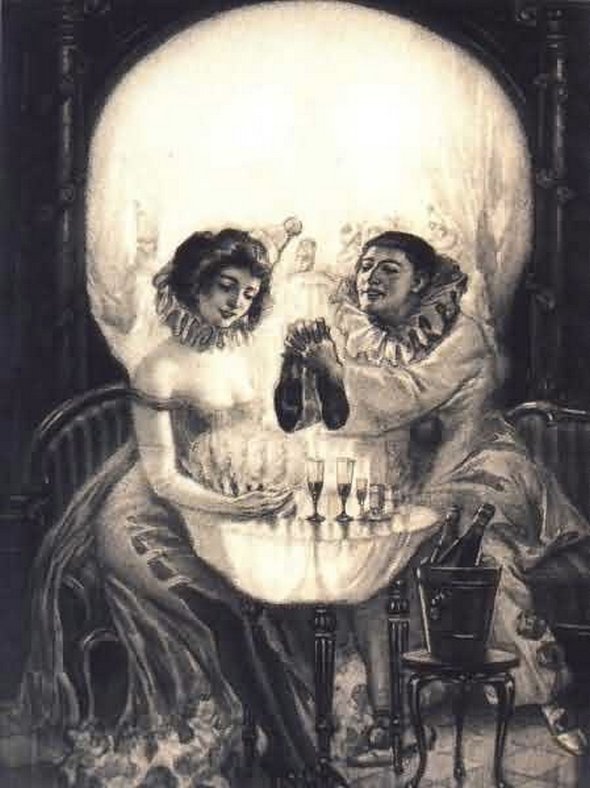This image is a cleverly crafted optical illusion, possibly created by AI. At first glance, it appears to be a black and white photograph of a giant skull. However, upon closer inspection, a subtle yellow tinge at the top suggests it may be a colorized version of a monochromatic image.

In the center of the composition, the skull's prominent features include two round eye sockets, a nasal cavity, and rows of teeth. The surrounding areas on the left and right are shrouded in black, while a grayish hue occupies the lower portion.

Shifting perspective reveals hidden details: Within the left eye socket, a woman's head emerges. She dons an Elizabethan collar and an off-the-shoulder dress, her arm extending around the skull's jawline, merging seamlessly into the gray background at the bottom.

Another figure appears on the right, their gender ambiguous. They, too, sport an Elizabethan collar and possibly tights or trousers. The lower part of their form also blends into the gray area.

A table materializes where the skull's teeth are, holding several wine glasses delicately placed between the teeth gaps. The figure on the right seems to be holding a bag, possibly offering it to the woman—an arm movement that aligns with the skull's nasal cavity. A small stool sits at the bottom right, supporting a bucket filled with wine bottles.

This artwork is an intricate and fascinating illusion, blending elements in such a way that initial appearances transform upon closer scrutiny.